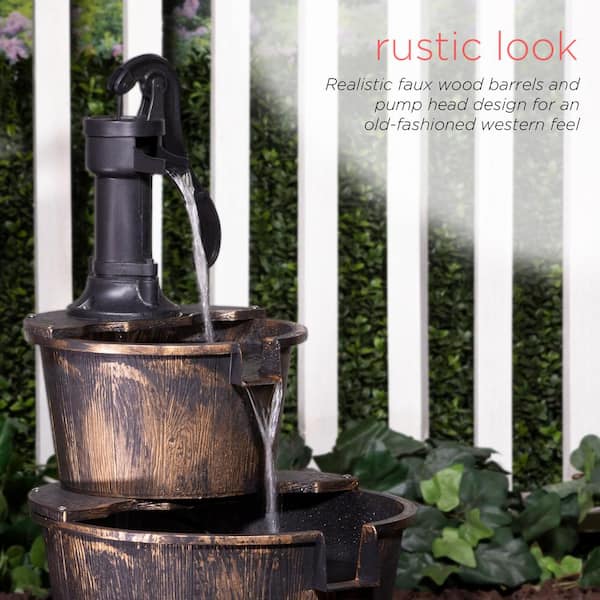This outdoor advertisement image features a rustic-style fountain prominently displayed on the left-hand side. The fountain consists of two stacked buckets with a realistic faux wood design, creating an old-fashioned Western feel. Water flows from a black metal faucet at the top, cascading from the smaller upper bucket into the larger lower bucket, producing a visible stream effect. The buckets are brown with dark grains, giving them a textured, woody appearance despite their metallic shine. In the upper right corner of the image, red and black italicized text states, "Rustic look, realistic faux wood barrels and pump head design for an old-fashioned western feel." The background showcases a white picket fence with some green hedges and vines near the lower right, adding a touch of lush greenery to the scene.